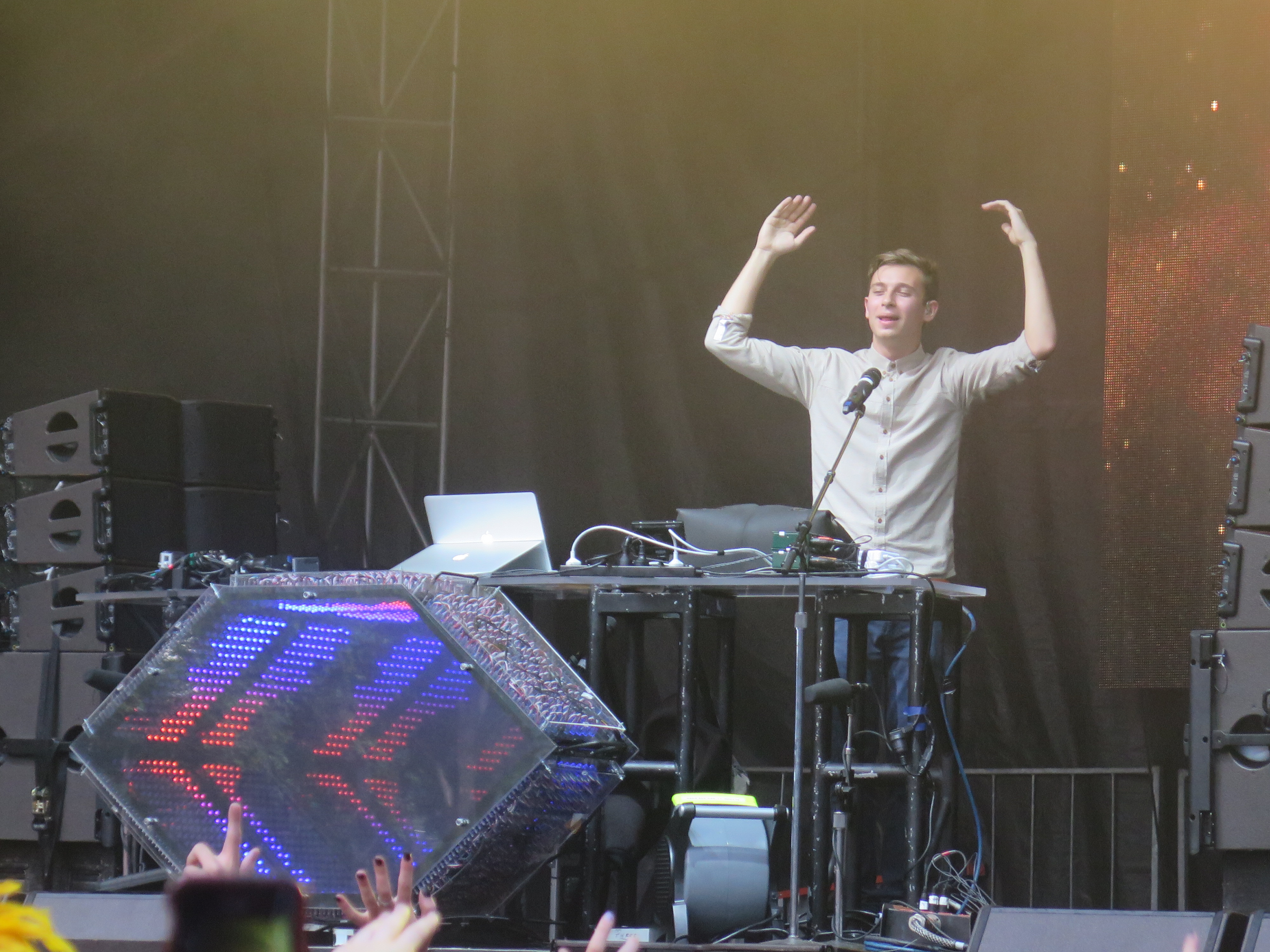The photograph captures a live concert scene featuring a white male performer standing behind a table on a stage, possibly a DJ. He is dressed in a white button-down long-sleeve shirt with rolled-up sleeves and blue jeans, sporting short brown hair. His eyes are closed and mouth open, as if in the midst of an expressive moment, with both hands raised in the air while speaking or singing into a microphone on a stand before him.

In front of him on the table are laptops and sound equipment, suggesting a DJ setup, although no traditional instruments are visible. The background features a solid black curtain, with additional stage elements such as scaffolding, stage pillars, big lights, and sound equipment visible off to the sides. To the left of the table, there is an arrangement of speakers stacked on each other, and to the right, parts of an LED screen displaying red and dark red hues can be glimpsed.

Adding to the ambiance, a hexagon or parallelogram-shaped object with LED lights glowing in various colors, including blue and red, is positioned in front of the table. The audience's presence is felt through their raised hands and phones captured in the foreground, indicating their engagement with the performance.